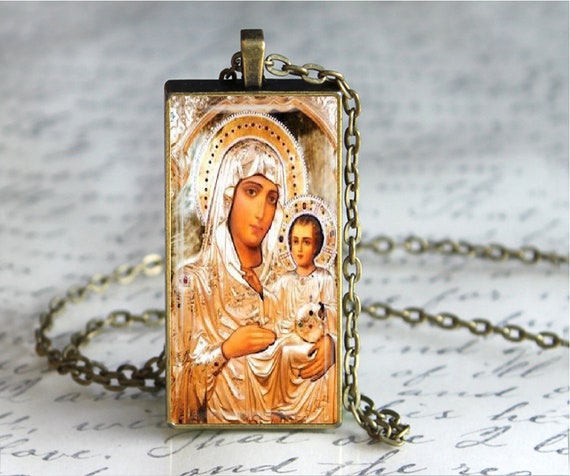The image features a detailed photograph of a rectangular pendant connected to a long, silver rope chain. The pendant showcases an illustration of Mother Mary holding baby Jesus, both adorned in silky or satin fabrics of pale golden or whitish hues. They are depicted with serious expressions, looking directly toward the viewer. Above them, there are gold, arc-like halos. The pendant, which appears to be around two inches tall, is placed against a page filled with cursive writing in black ink, adding a classic and sophisticated backdrop to the religious-themed jewelry piece. The overall color palette of the image includes beige, tan, white, and touches of brown, further emphasizing the serene and sacred ambiance.